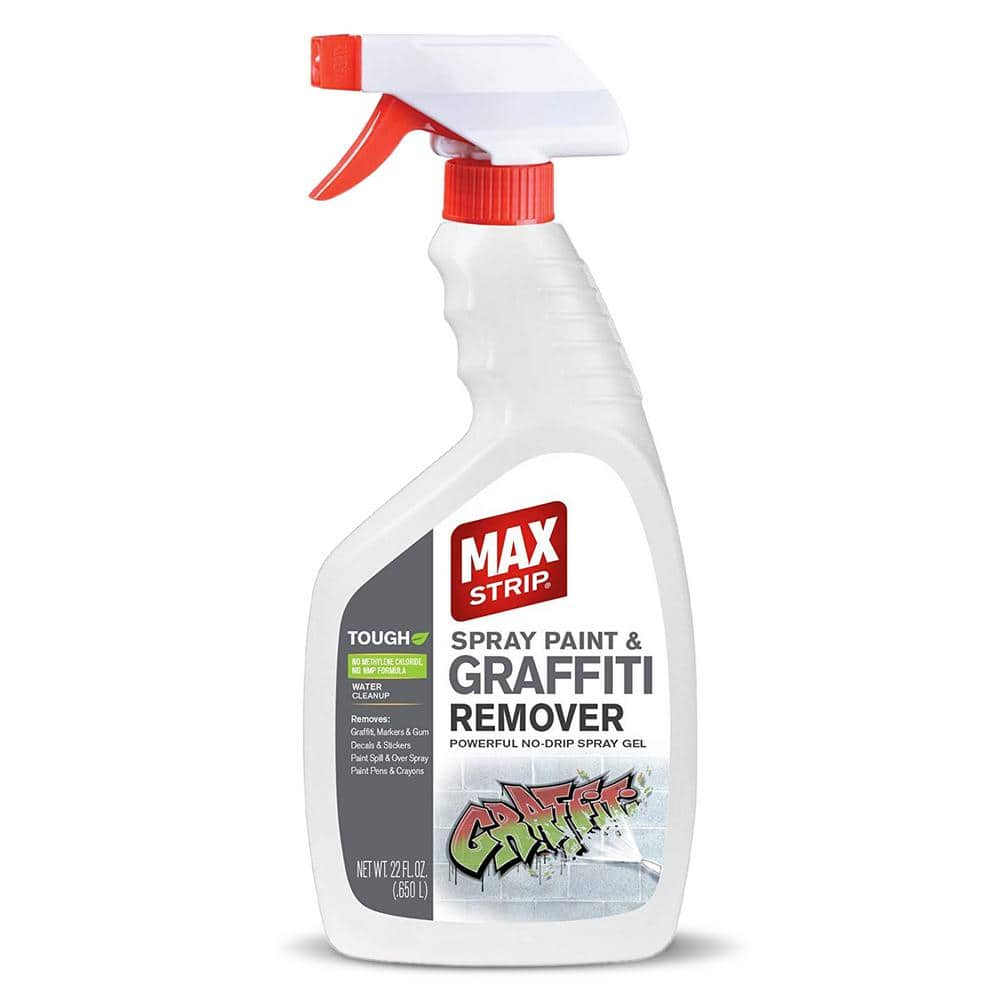This promotional product photo features a close-up of a white plastic spray bottle of "Maxstrip" spray paint and graffiti remover. The bottle sports a red spray trigger, nozzle, and handle, while the rest of the bottle is white. The label on the front is prominently adorned with a red square background featuring the "Maxstrip" logo in white lettering. Below this, in gray text, it reads "Spray Paint and Graffiti Remover" alongside the description "Powerful No Drip Spray Gel." The label also includes an image of a wall with multicolored graffiti in red and green. To the left of the graffiti image, the word "Tough" is printed. The bottle contains 22 fluid ounces (650 ml) of the product, as indicated in white text. The clean, white background of the image suggests it is intended for online retail use.